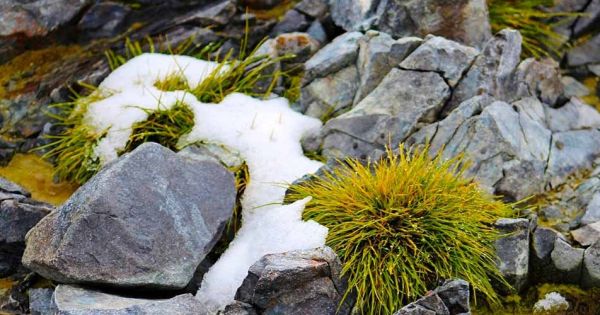The photograph captures a rugged natural scene with a striking composition of jagged gray and brown rocks interspersed with patches of green and yellow spiky plants. On the left side, there's a dominant gray rock accented with purple, flanked by a smaller black rock. In the top left corner, a cluster of darker rocks is tinged with rusty, orangey-brown hues. Below these rocks lies a band of brown foliage. Adjacent to this foliage and sweeping towards the bottom center is a patch of snow, interrupted by various plants poking through. This snow patch extends longitudinally between a large rock on the left and a series of both large and small rocks on the right. Just to the right of the snow, a significant, fuzzy plant with light green spikes mixed with hints of orange stands out, partially covered by a thin layer of snow. Further to the right, a mound of gray rocks meets a clearing where another green spiky bush resides. This bush appears unscathed by the snow except for a faint dusting on its tips. The overall scene is set against the backdrop of daytime, enhancing the intricate details of this cliff-edge environment.